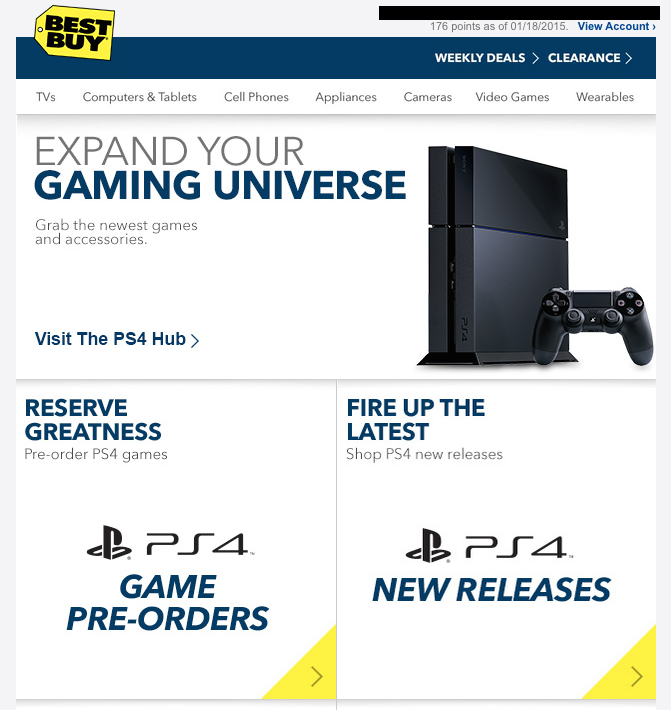Here is a cleaned-up and detailed descriptive caption for the image:

---
The image is a webpage screenshot from the Best Buy website. In the top left corner, the distinctive Best Buy logo is displayed, resembling a yellow price tag outlined in black, complete with a hole for a string located in the middle left area. The logo prominently features the words "BEST BUY" written in bold, black, capital letters.

Directly beneath the logo, a navy blue horizontal rectangular section draws attention. Positioned towards the right-hand side of this navy blue area are the words "WEEKLY DEALS” and “CLEARANCE,” each in bold, white, capital letters separated by greater-than signs (>).

Following this section, a white background hosts a series of product categories listed in gray font from left to right, including: TVs, Computers & Tablets, Cell Phones, Appliances, Cameras, Video Games, and Wearables.

Below this, a horizontal promotional image spells out in all capital letters, "EXPAND YOUR GAMING UNIVERSE" with the phrase "Expand Your" in gray and "Gaming Universe" in navy blue. Underneath, the gray text reads, "Grab the newest games and accessories." At the bottom of this promotional section, navy blue text states, "Visit the PS4 Hub >".

On the right-hand side of this section, a black game controller and a black gaming console unit are featured.

The next segment of the image contains two vertical rectangular areas. The first rectangular area has the bold navy blue text in the upper left corner stating, "RESERVE GREATNESS." Beneath it, in gray text, is the phrase "Pre-order PS4 games." Lower down in this section, there is a "PS4" logo, and at the bottom in bold navy blue capital letters, the text reads "GAME PRE-ORDERS," all set against a white background with a yellow triangle containing a greater-than sign (>) in the lower right corner.

The final section features a navy blue header with bold, all-capitalized text reading "FIRE UP THE LATEST." Below this, the text states in gray, "Shop PS4 new releases" followed by another "PS4" logo. At the bottom of this area, the text in bold, navy blue, capital letters reads "NEW RELEASES," with the same yellow triangle and greater-than sign (>) in the lower right corner.
---

This detailed description should give a clear and comprehensive overview of the image content.